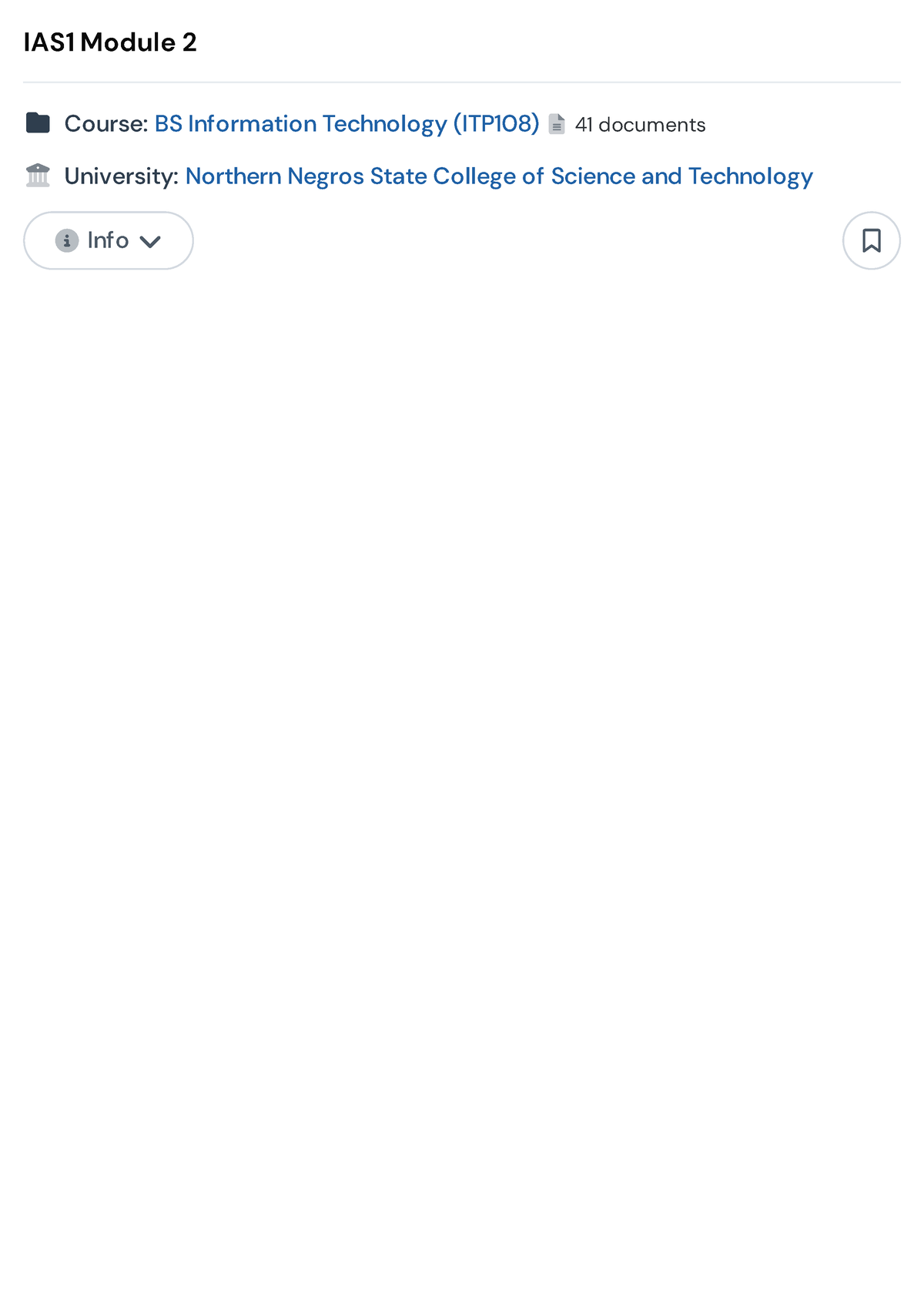This small image, likely a screenshot from a smartphone, features a blue and white interface with both blue and black text. 

At the top, bold black text reads "IAS1 Module 2," which is followed by a light gray horizontal dividing line. Below, there are two lines of text. The first line includes a black folder icon next to the word "Course:" in black. The text continues in blue, stating "BS Information Technology" with "ITP108" in parentheses. Following this, a page icon is displayed, along with the phrase "41 documents" in black.

The second line features a school icon next to the word "University" in black, followed by blue text reading "Northern Negros State College of Science and Technology." Below these lines, there is a drop-down button labeled "Info," and on the far right of the line is a bookmark symbol.